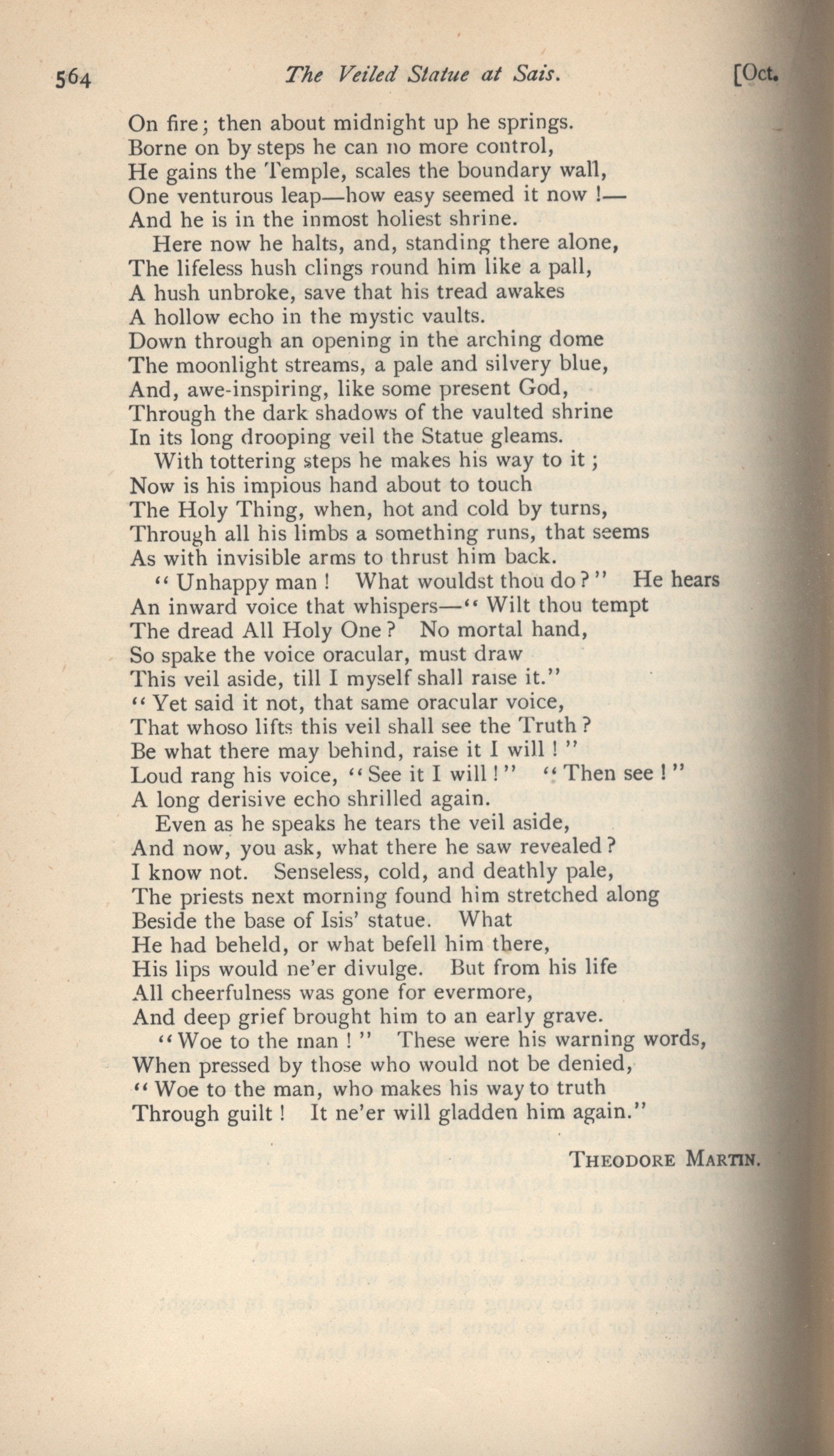This image depicts a weathered and yellowed page from an old book, suggesting considerable age and usage. The page number, 564, is clearly indicated in italicized print in the upper left-hand corner. In stark black at the top center is the title, "The Veiled Statue at Sais," with "Sais" spelled S-A-I-S. The upper right-hand corner features the abbreviation for the month of October, noted as "[OCT.]." The main body of the page is densely packed with prose, consisting of approximately six to seven paragraphs of small, black type. A light shadow, presumably from the book’s spine, is cast along the right edge of the page. Towards the bottom right is the author’s name, THEODORE MARTIN, prominently printed in all capital letters. The page concludes with a small area of blank space, indicating the end of the text.